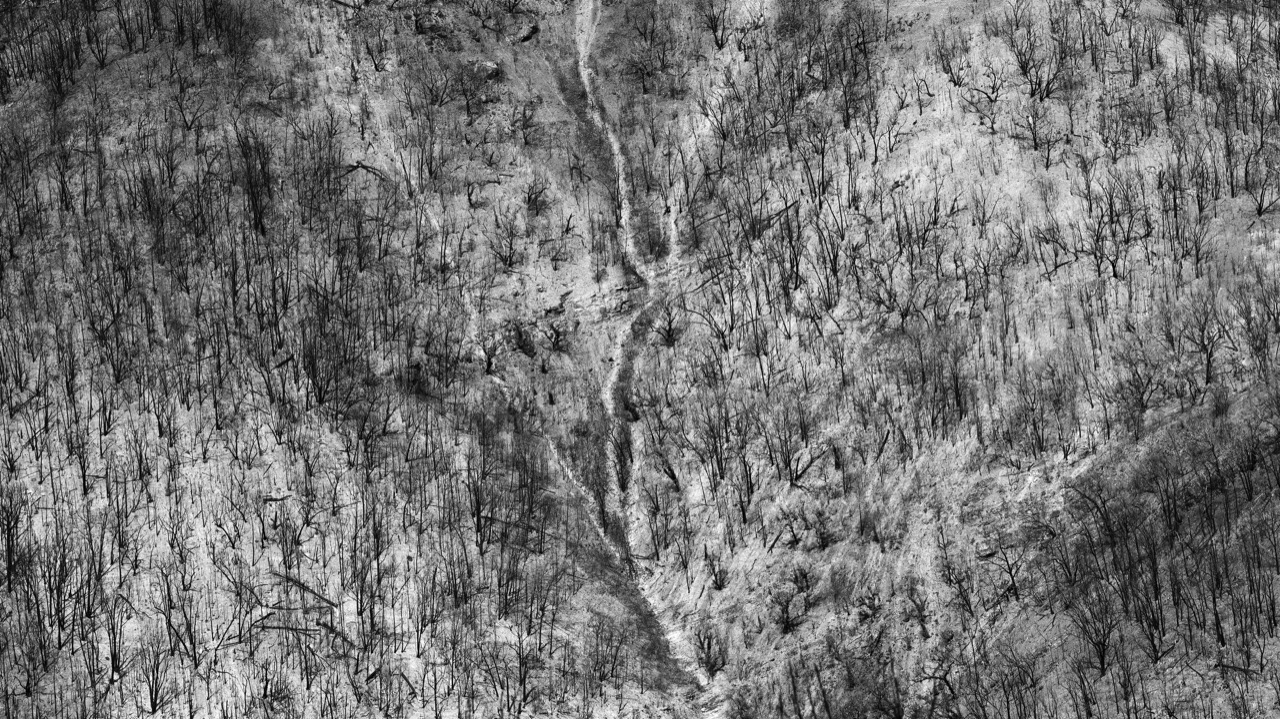This black and white image features an aerial view of a dense, barren forest, capturing a stark and desolate landscape. The scene looks as though it has been sketched with a pencil, emphasizing the grim and intricate texture of the withered trees, which have no leaves. Their dark, skeletal forms contrast sharply against the lighter ground, suggesting either a bleak winter or the aftermath of a forest fire. A dried-up river or stream zigzags through the center of the image, from top to bottom, adding to the overall feeling of desolation. The uniformly gray tones of the photograph further accentuate the eerie, lifeless atmosphere, with the high vantage point, possibly 500 to 700 meters above, giving a comprehensive view of the dense, stick-like trees crowding the desolate hillside or mountain terrain.